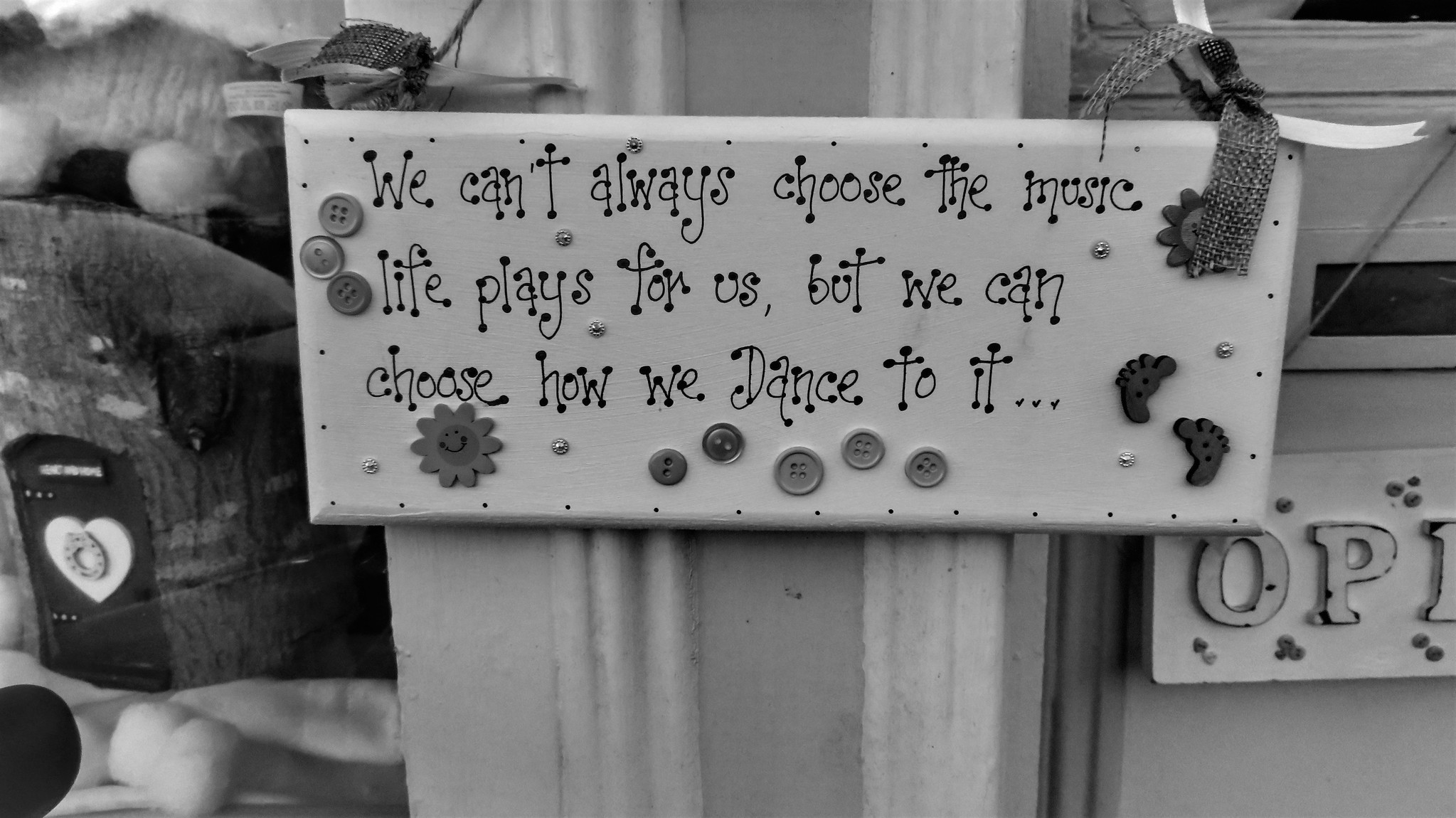In this black and white photograph, a charming, artsy ceramic plaque hangs prominently in front of a door. The plaque is secured by wires adorned with small, cloth bows on each side, giving it a delicate, handmade appeal. The sign itself bears an uplifting message in a playful, dotted font that reads: "We can't always choose the music life plays for us, but we can choose how we dance to it." Enhancing its crafty design, the plaque features several buttons, a footprint pattern, and decorative elements that resemble a sun and possibly flowering motifs. The texture and detailed craftsmanship, including the twine cloth ribbons on the edges, add to its whimsical nature. To the left of the plaque, part of another sign is visible with the letters "O, P, E," while on the right, a window exposes a glimpse inside the building where a couch can be seen. The overall composition creates a quaint and inviting scene despite its monochromatic tone.